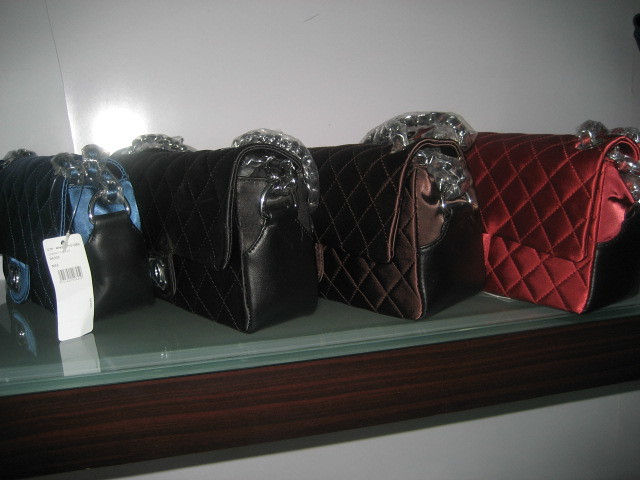The photograph captures four luxurious, medium-sized pocketbooks, neatly arranged on a wooden display shelf against a white wall. Positioned at a slight angle, each one showcases both its front and right side, with the fronts uniformly facing left. The pocketbooks, crafted from textured, high-quality materials, exhibit a sophisticated design that features rugged chain handles encased in plastic, leather-like loops for attaching belts, and woven fabric with a diamond pattern. The first pocketbook sports a striking blue and black color scheme and still carries a price tag. The second is entirely black, followed by a brown one. The fourth and final pocketbook is a vibrant, shiny red. The combination of their materials, colors, and presentation underlines their status as designer, luxury items.